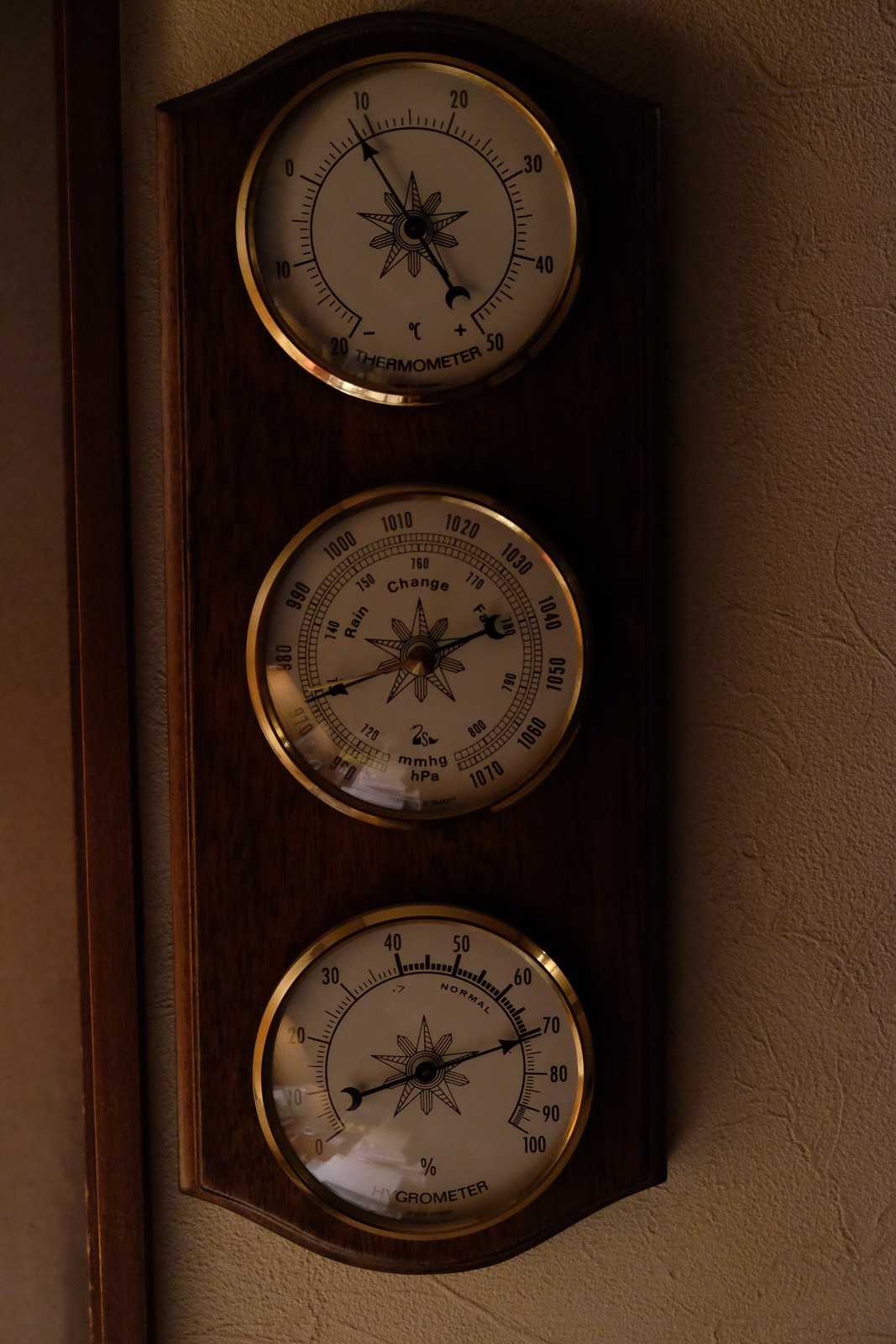The image showcases a wooden panel mounted on a wall, featuring three distinct measuring instruments arranged vertically. At the top of the panel is a thermometer, clearly labeled and calibrated to measure temperatures ranging from -20 to 50 degrees. The middle instrument is a barometer, identified by the label "Barometer" and its scale which is measured in millimeters of mercury (mmHg), extending up to 1070 mmHg. The third and bottom device is a hygrometer, designed to measure humidity levels from 0 to 100%. Each instrument has a white face, encased in a shiny chrome frame, contributing to a cohesive and polished appearance. The wooden panel that houses the instruments is mounted against a white or off-white wall and is bordered by a similarly colored vertical wooden strip, adding a harmonious, rustic touch to the presentation.